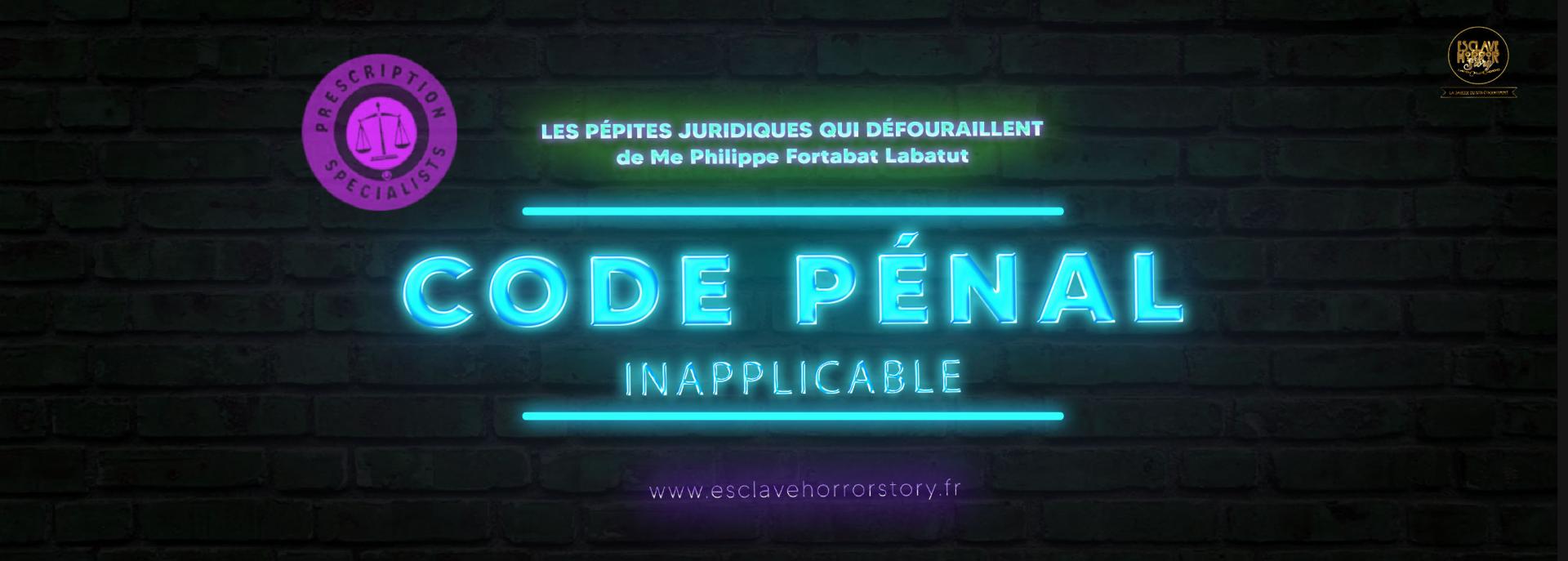The image features a digital neon banner set against a very dark gray, nearly black, brick wall, giving it a dimly lit ambiance. Dominating the upper left corner is a circular purple logo, showcasing a set of old-fashioned scales, flanked by some text that isn't clearly legible. The central portion of the banner prominently displays the text "Code PÉNAL Inapplicable" in large, neon blue letters, conveying the main message in French. Surrounding this main text, additional words are present in smaller, fluorescent green print, but they're difficult to decipher. Near the bottom, a web address glows in purple light. The overall image employs a palette of black, purple, neon blue, and fluorescent green, contributing to its striking and vivid visual impact. The design likely functions as an advertisement or sign, potentially for legal or prescription services, given the scales logo and the bold proclamation in the center.